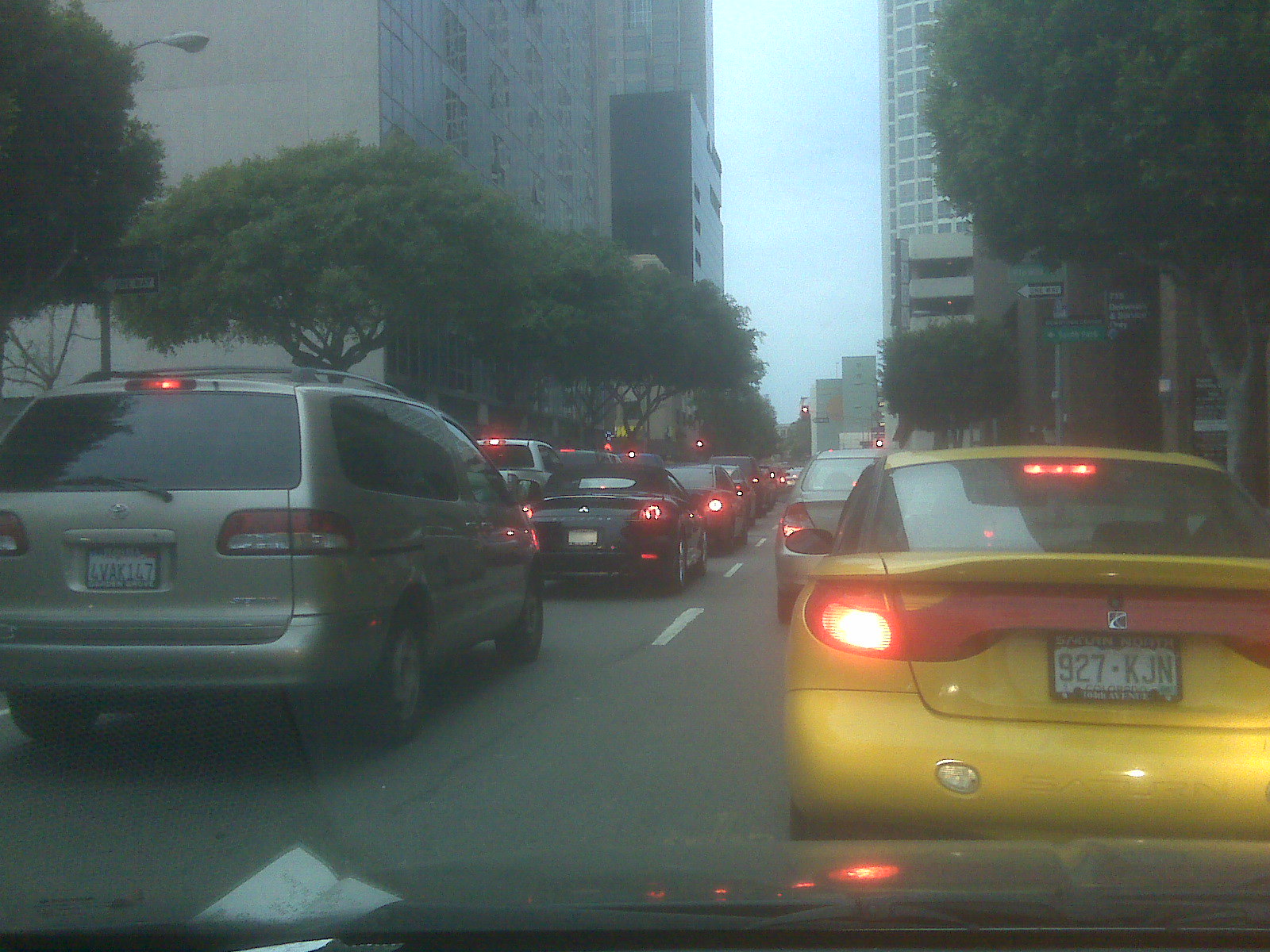This photograph, taken from within a vehicle stalled in heavy traffic, depicts a congested urban street. Stretching into the distance, the traffic remains bumper-to-bumper up to the visible streetlight, which glows red approximately a block and a half away. Every vehicle's taillights and brake lights illuminate the scene, except the minivan directly ahead, whose brake light is positioned on top of its cargo door. Both sides of the street are lined with trees, their lush canopies creating an umbrella-like effect over this treelined block. Flanking the roadway are towering high-rises, likely office buildings, contributing to the urban skyline. It's a hazy yet daylight-filled day, obscuring the full extent of the high-rise structures. The street itself appears to be a three-lane thoroughfare, though there may be additional lanes out of the frame, with a cross street intersecting the current view.